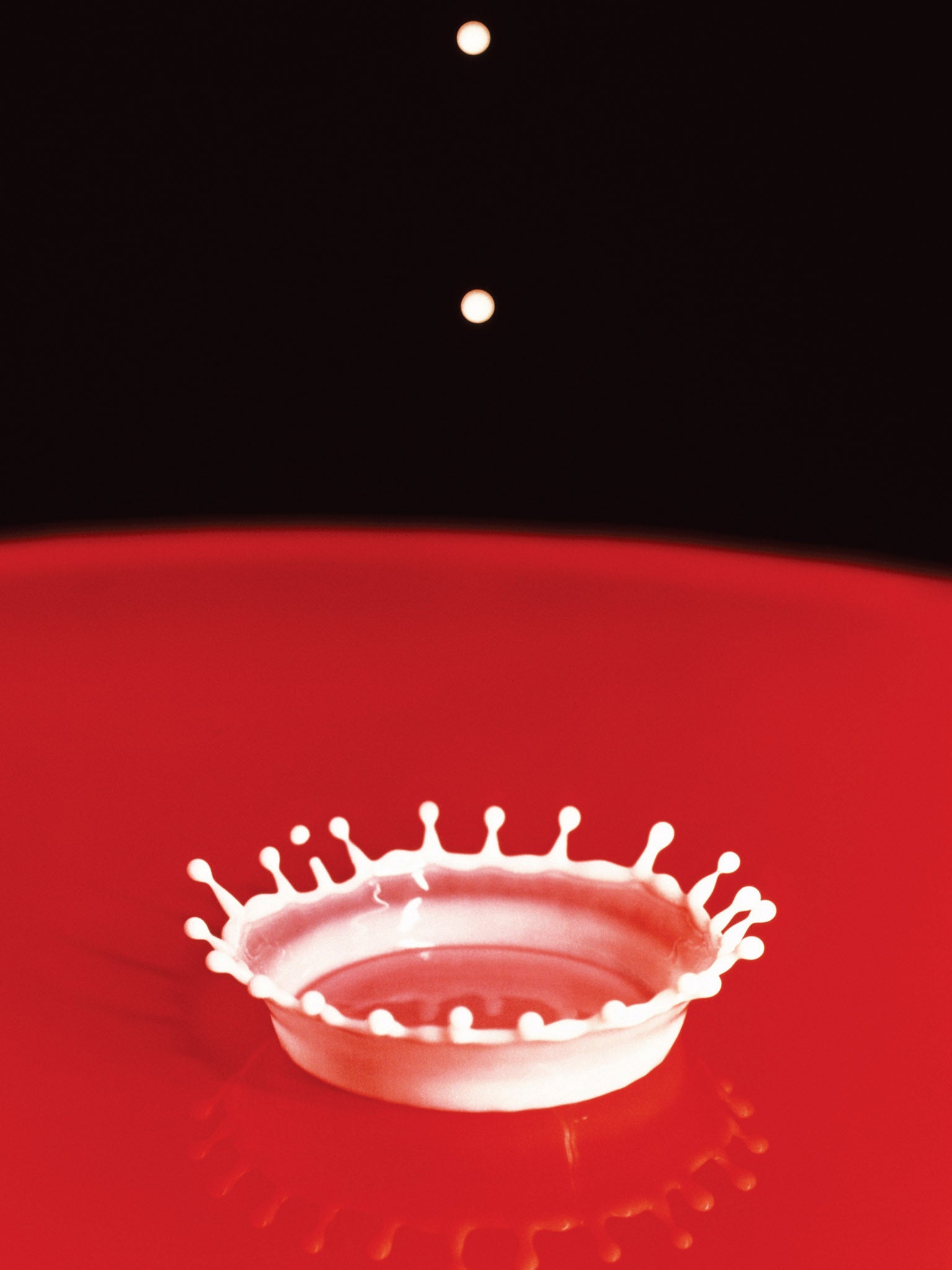The image is a tall rectangle, dominated by a bright red, glossy, round surface at the bottom, which appears to be a close-up of a table. In the center of this red table, there's a striking white ring that resembles a splash of milk or dripping candle wax, frozen at the point of impact. This splash forms a spiky crown-like shape with small white balls atop each spike, reminiscent of a royal crown. The background above the red table is entirely black, punctuated by two small white dots aligned vertically, resembling buttons on a black shirt or distant stars. The overall scene evokes the moment of a milk drop hitting the table and bouncing back up, captured in a vivid, almost surreal display, with additional milk drops visible suspended in the dark background.